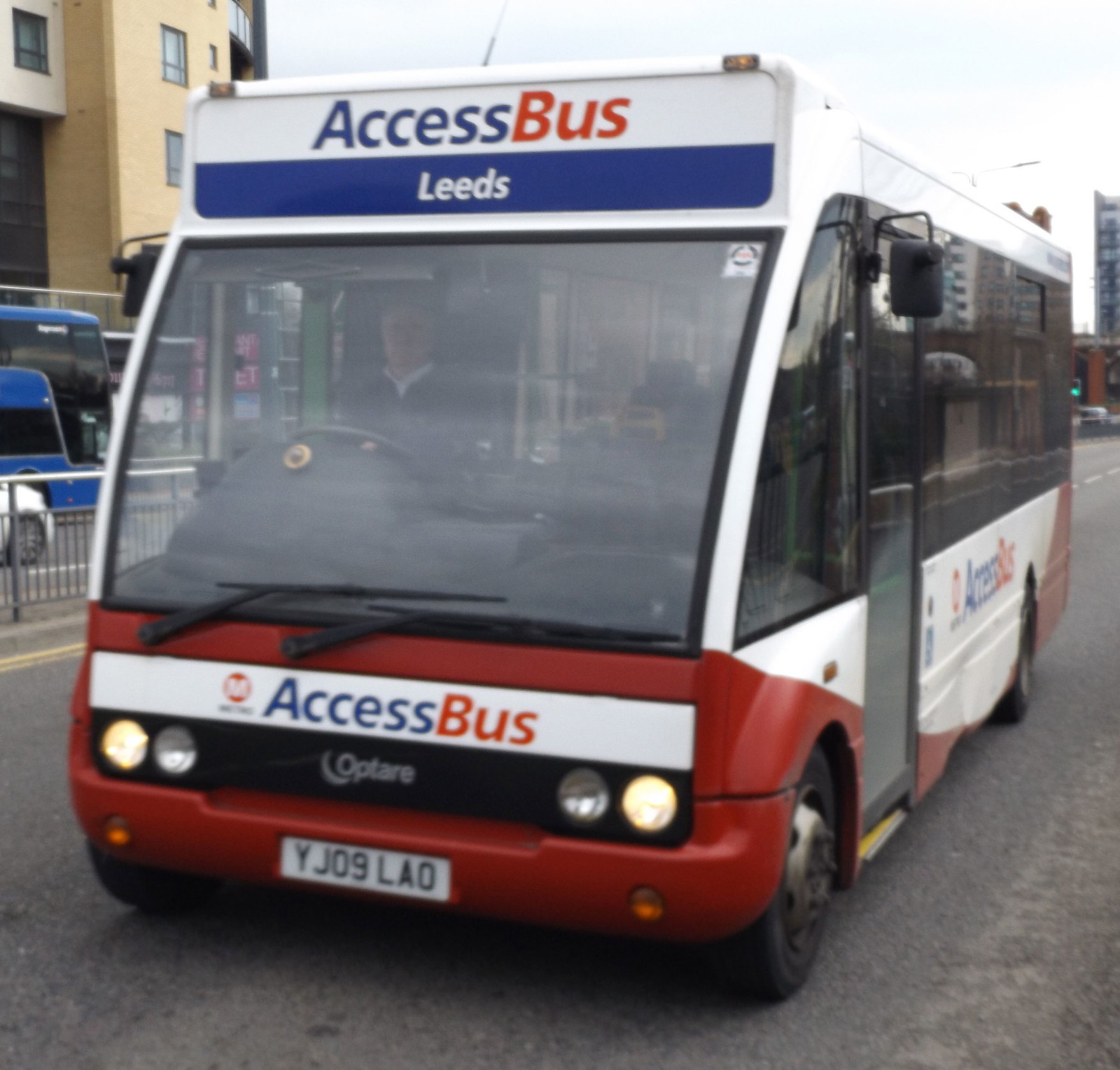The image depicts a city street scene featuring an Access Bus adorned in blue, red, and white colors. Above the windshield, a sign displays "Access Bus" in blue on a white background, followed by "Leeds" in white against a blue background. Below the windshield, the bus again features "Access Bus" in a similar format, while beneath that is the manufacturer's name "Optare." The bus's license plate reads YJ09LAO. The vehicle is currently driving on a two-lane road, with visible yellow lines to its left and behind. Part of the sky is seen at the top of the image, showing blue and white hues. Surrounding the bus, there are additional buses and cars, with nearby pavements and a fence. In the background, various buildings, possibly housing or apartments, can be spotted. No passengers are visible inside the bus.